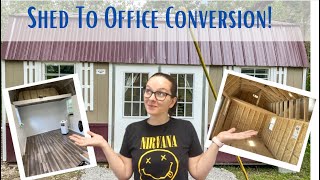The image features a woman standing centrally, wearing a black t-shirt with "Nirvana" written in yellow and a smiley face with X's for eyes beneath the text. Behind her is a small shed, identified as such by the blue text at the top of the image that reads "Shed to Office Conversion!" Superimposed upon the main photograph are two smaller inset images. The image on the left shows the unfinished interior of the shed, highlighting bare walls and flooring. The image on the right displays the completed renovation, featuring finished walls and flooring. The woman, a white woman with glasses, holds her hands up as if presenting the transformation depicted in the inset photos.